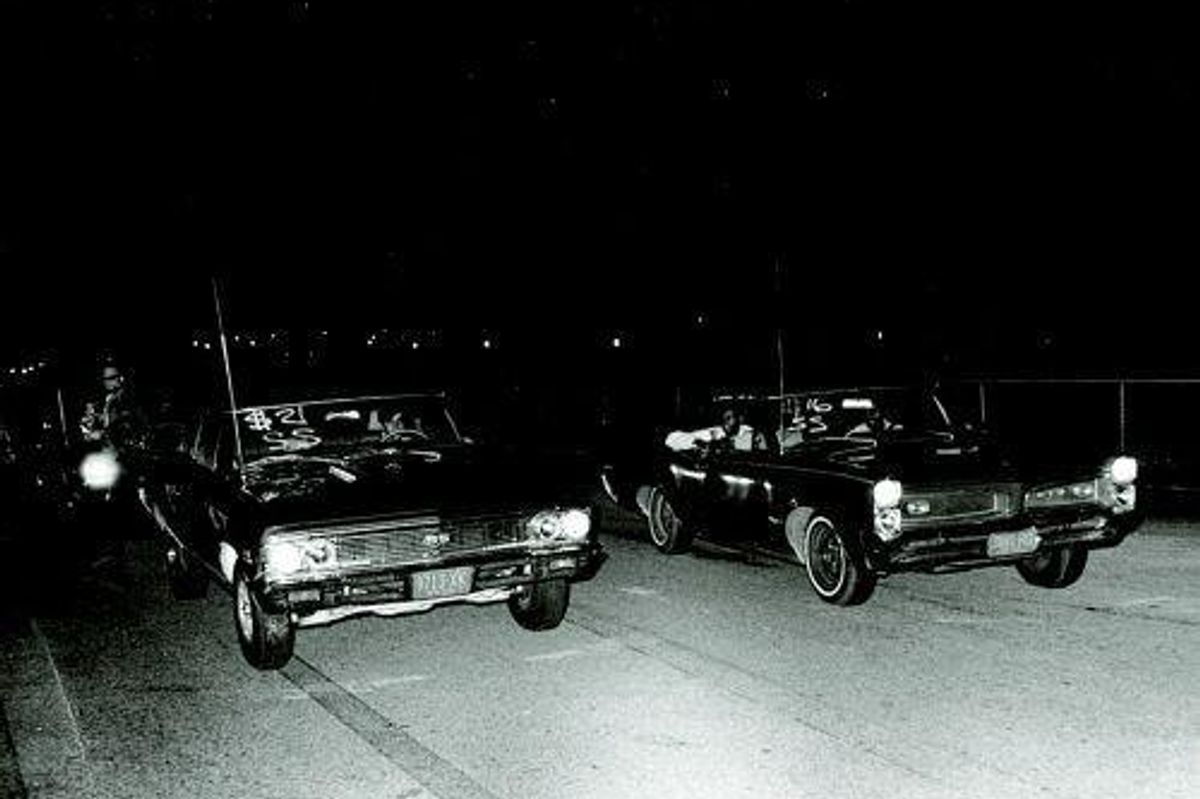In this black and white nighttime photograph, two cars, likely from the 60s or 70s era, are positioned side by side in a racing stance on an asphalt street. Both vehicles have their headlights on, illuminating the dark scene around them. The street surface shows tire marks and stains, indicative of frequent racing activity. The car on the left features a distinct marking on its windshield—a dollar sign followed by the number 21 and the letters "SS." A man is seen standing next to this car, while another person is walking behind it, partially visible in the background. The car on the right also has "SS" on its windshield, with a passenger visible in the vehicle’s right seat. The photograph is dominated by a pitch-black sky, with a few distant lights providing minimal background illumination.